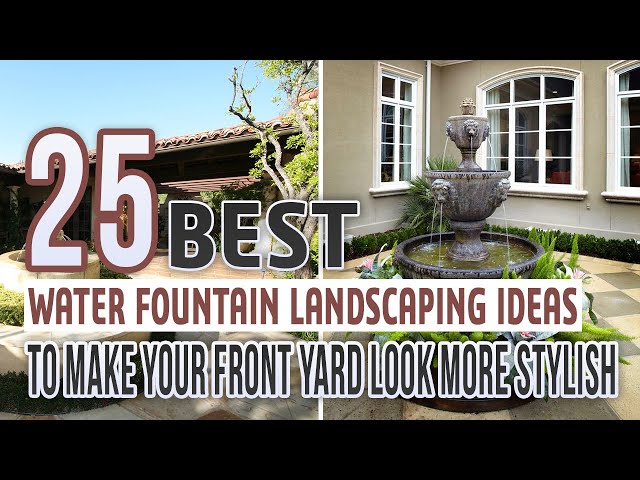The image is a horizontal rectangular photograph with a black border on the top and bottom. It features two smaller photos side by side. The left photo shows a house with a light gray exterior and white window frames, a small fountain in the foreground, a blue sky, and trees with bright green leaves. The right photo is a close-up of a multi-tiered, dark brown water fountain adorned with lion heads, water flowing from their mouths. Centered between the two photos, there is text that reads, "25 best water fountain landscaping ideas to make your front yard look more stylish." The number "25" is in white with a brown border, "best" is in all capital letters in black with a white border, "water fountain landscaping ideas" is in brown, and "to make your front yard look more stylish" is in black with a white border. The overall setting appears to be an elegant exterior with lush greenery and stylish water features enhancing both the front and backyard of a house.